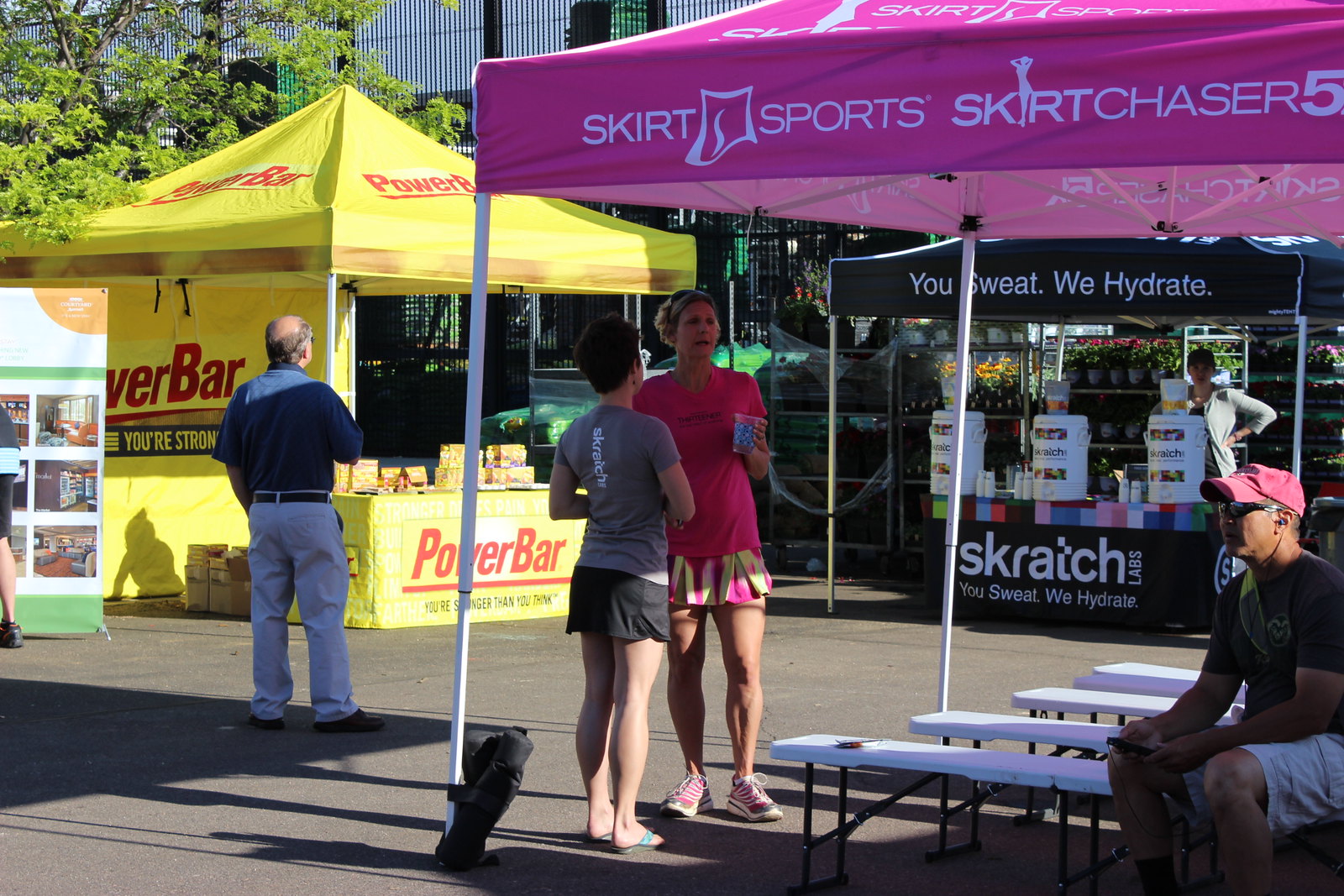The photograph captures an outdoor event venue featuring multiple sponsor booths in a somewhat sparse setting. On the left side, there's a yellow booth with a triangular top labeled "Power Bar." At the front of this booth, a table displays some yellow boxes, and a man stands in front, staring at the setup. To the right in the immediate foreground, another booth features a pink canopy with "Skirt Sports Skirt Chaser 5" printed on the roof. Further back on the right side, a black booth prominently displays the slogans "We Sweat, We Hydrate" and "Skratch" on the top and front, respectively. In front of this booth, there are three white buckets of drink. The area appears to be relatively quiet with only a few people milling about, suggesting that the event has not yet fully started.